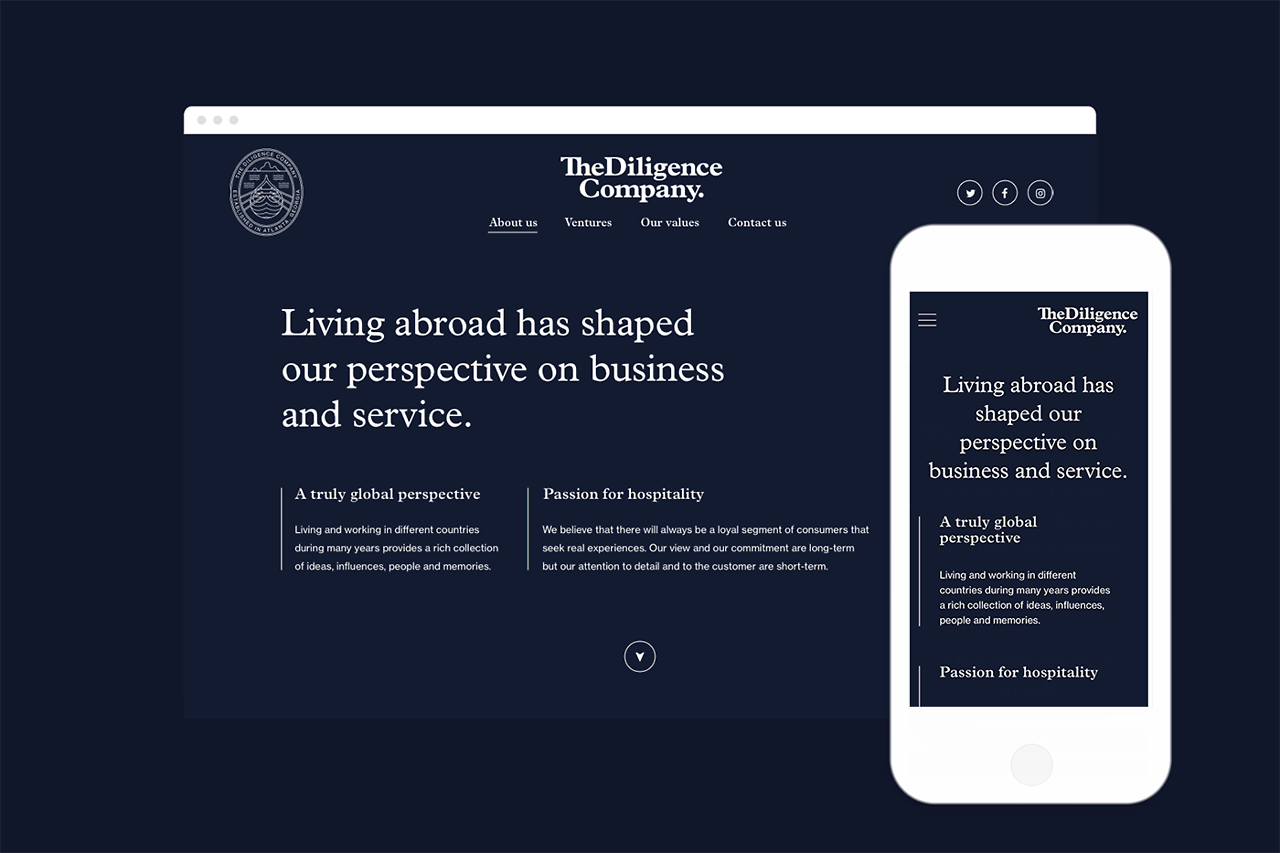The image features a black screen with white text showcasing the website of "The Diligence Company." At the top, there are four tabs labeled "About Us," "Ventures," "Our Values," and "Contact Us." Below the tabs, a message reads, "Living abroad has shaped our perspective on business and service, offering a truly global outlook. Years of living and working in different countries have provided a rich collection of ideas, influences, and memories." This text is quite small. 

Further down, there's a section titled "Passion for Hospitality," which states: "We believe there will always be a loyal segment of consumers seeking authentic experiences. Our view is rooted in commitment, long-term dedication, and a meticulous attention to customer detail, both in the short-term and long-term."

To the right side of the image, the same screen is displayed on a white smartphone, mirroring the website's interface.